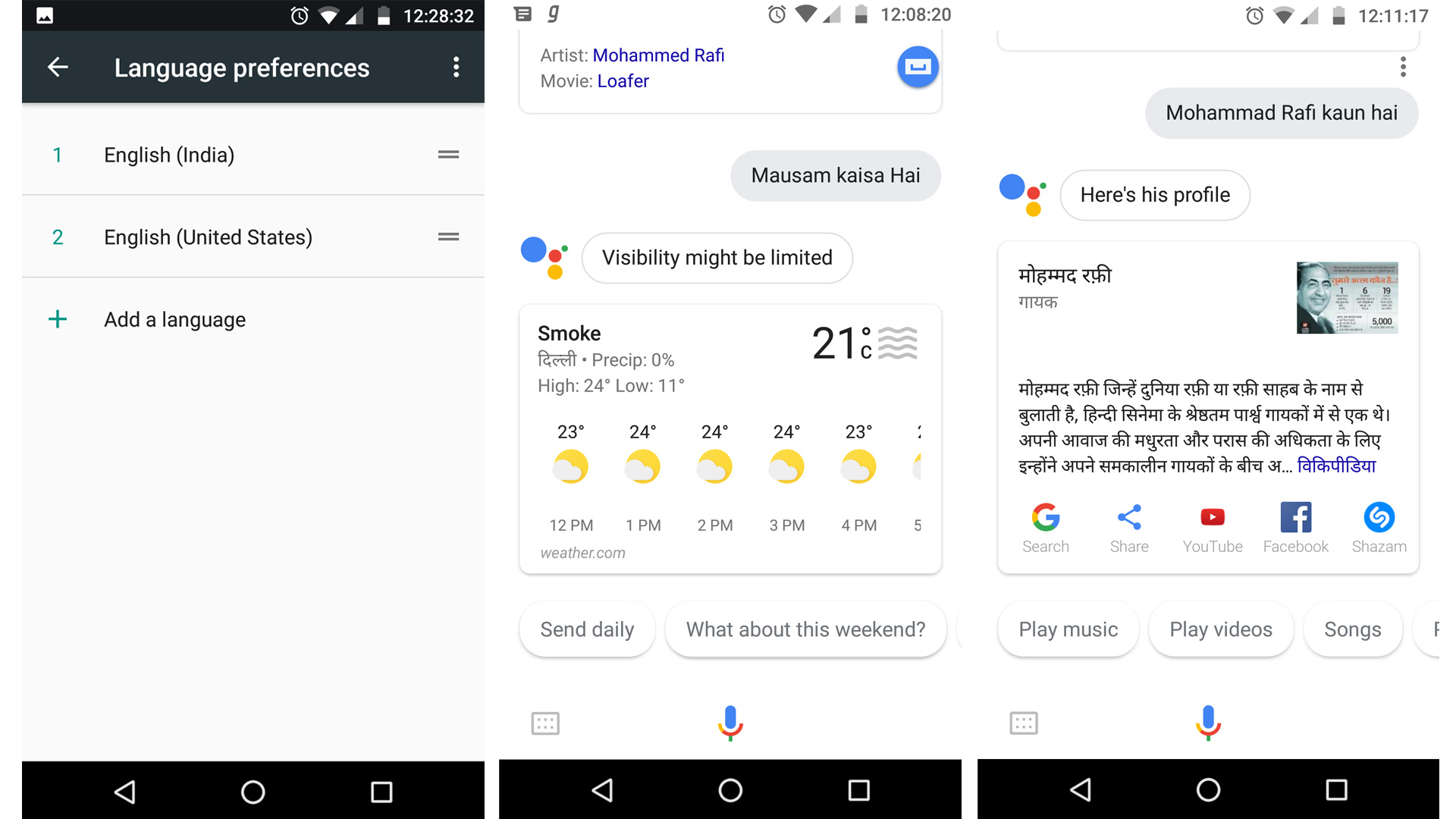The screenshot image on the left displays a mobile interface with various details. At the top, the battery indicator shows 2 out of 4 bars remaining. The time is displayed as 12:28 and 32 seconds. Below the time, there's a section labeled 'Language Preferences': 
1. English (India)
2. English (United States)
There is also an option to 'Add a language.'

On the right side, the artist Mohamed Rafi is referenced, specifically from the movie "Loafer." A text box contains the phrase "Masam-Kaiza-Hi." Underneath, there's a notice that reads: "Visibility might be limited." The weather details indicate it's smoky with a temperature of 21 degrees Celsius, no precipitation, a high of 24 degrees, and a low of 11 degrees. Below this, a prompt suggests: "Send daily updates. What about this weekend?"

To the right, another text box lists "Mohamed Rafi Khan-Hi" and mentions, "Here's his profile," followed by a box containing text in Hindi. Below this, there are icons or options for 'Search,' 'Share,' 'YouTube,' 'Facebook,' and 'Shazam.'